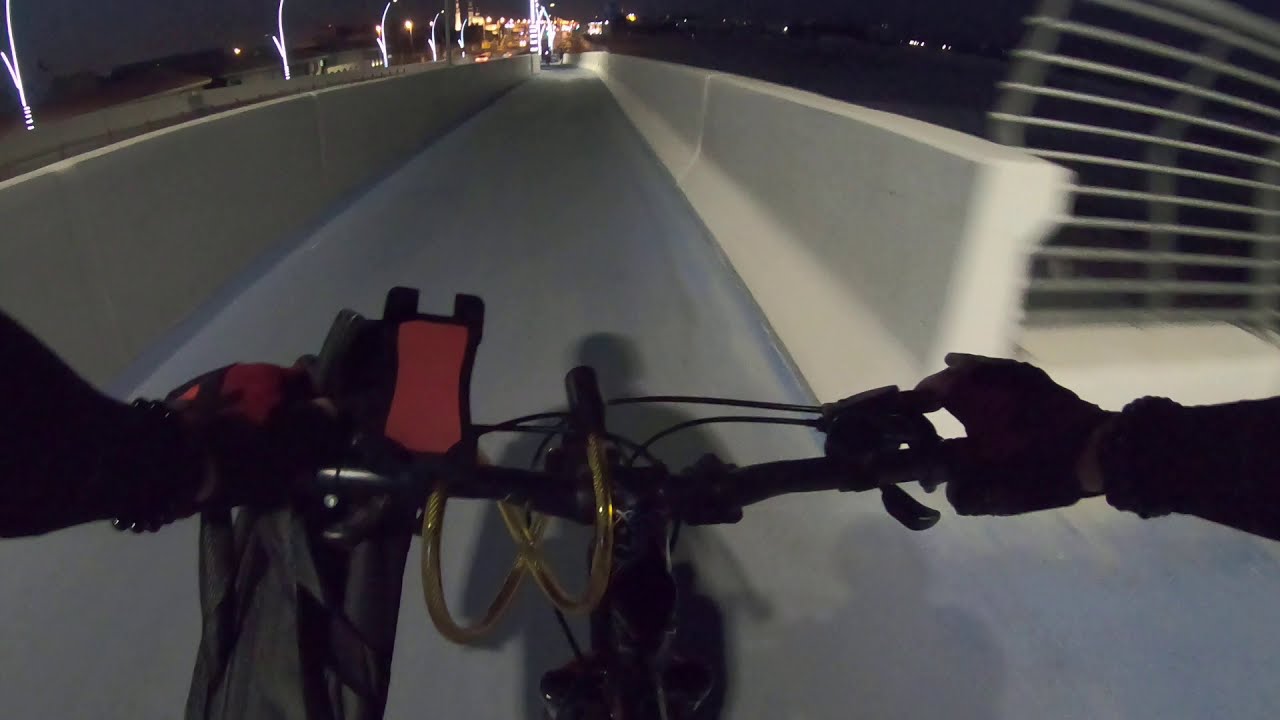In this nighttime GoPro footage, a cyclist is seen riding a mountain-style bicycle along a bridge or road with a concrete retaining wall on either side, blurred to show motion. The rider, likely male and wearing black gloves and a dark outfit, grips the handlebars, which feature a lock wrapped in gold-colored tubing and auxiliary equipment including a smartphone mount with a red center. The cyclist's shadow stretches ahead on the gray asphalt pavement under the illumination of overhead streetlights. In the distance, city lights and various structures are visible, framing the dark, scenic night ride.